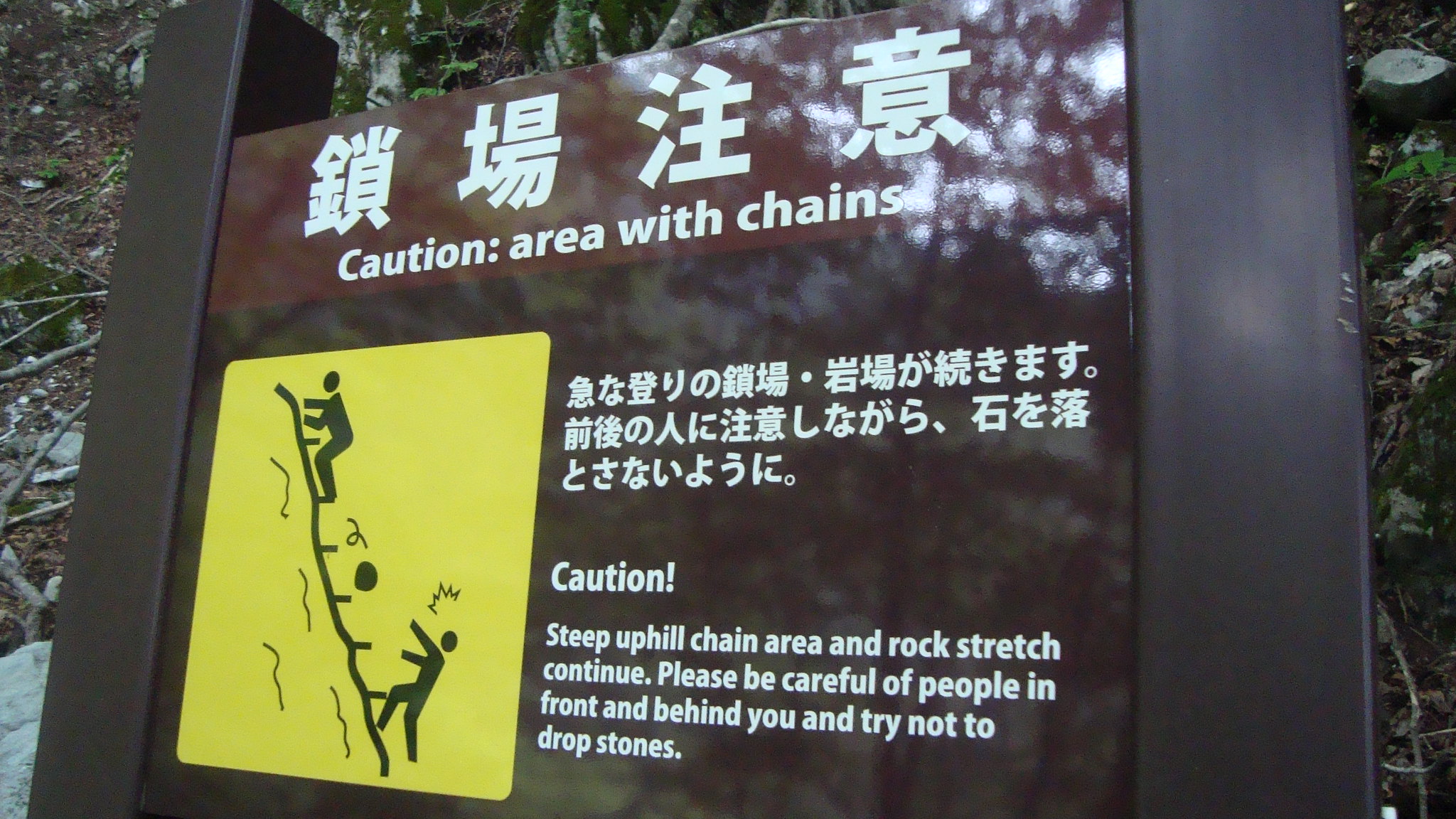The image depicts a brown signpost situated in a wooded outdoor area, likely near a climbing trail or a steep hike. The sign features multiple warnings both in Asian lettering, likely Chinese, and in English. At the top, four Chinese characters in white stand out prominently against the brown background. Below them, English text reads: "Caution: Area with chains." Further down, a yellow warning graphic illustrates two climbers, one of whom is at risk of being struck by a falling rock, emphasizing the need for caution. Adjacent to this image, additional Chinese characters are visible, reinforcing the warning. The English text proceeds with detailed instructions: "Caution! Steep uphill chain area and rock stretch continue. Please be careful of people in front and behind you, and try not to drop stones." The sign is mounted on dark brown posts, and although the material appears glass-like and reflective, it shows an overall blend of browns, whites, yellows, and some greens and grays from the surrounding foliage, indicating a forested hill setting, likely on a sunny day. The sign appears relatively new, contributing to the vibrant and colorful visual aspect of the scene.